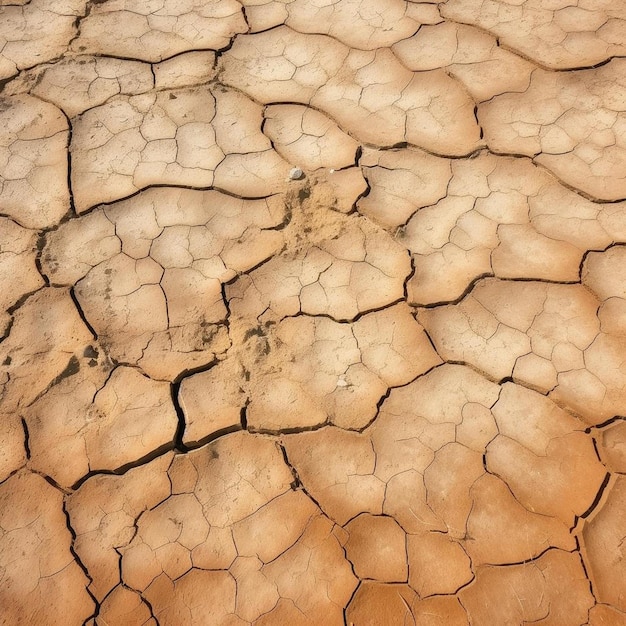This aerial photograph captures an expanse of arid, parched land featuring a spectrum of beige, tan, and cream hues. The terrain is heavily cracked, reflecting the extreme dryness and lack of hydration. Darker, wider cracks snake through the desolate landscape, indicating areas of potential instability and danger. Surrounding these prominent fissures are myriad thinner, lighter cracks that create a complex, intricate web across the hardened earth. In the center of the image, small piles of sand disrupt the otherwise uniform expanse, hinting at movement and activity. The overall appearance is both orderly and chaotic, characterized by the varying sizes and depths of the fissures.